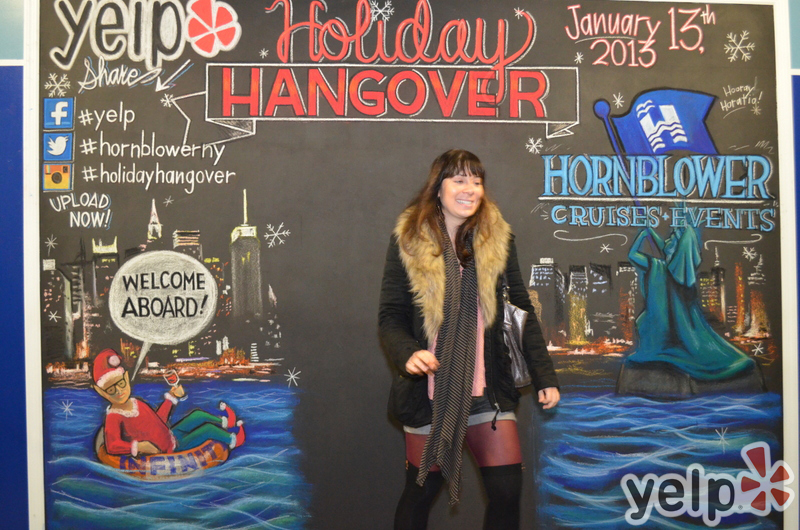The image depicts a woman standing in front of a large black chalkboard-like wall, adorned with intricate chalk illustrations. At the top of the board, in red cursive letters, it reads "Holiday Hangover," with the event date "January 13, 2013" inscribed nearby. On the left side of the chalkboard, there's a whimsical illustration of an elf wearing a Santa hat, floating in a life raft and holding a glass of wine, with a speech bubble above him that says, "Welcome aboard." To the right, there is a chalk rendition of the Statue of Liberty, holding a blue flag with an 'H' on it, alongside the logo for "Hornblower Cruises & Events." A city skyline can be seen faintly in the background. Additionally, the Yelp logo is visible on the top left corner of the chalkboard. The woman, who is smiling, has long brown hair and is dressed warmly in a black coat with a faux fur collar, a long gray and white scarf, a miniskirt with tights, and over-the-knee black boots. The overall setup suggests it's a spot for attendees to take selfies at an event hosted by the cruise line.